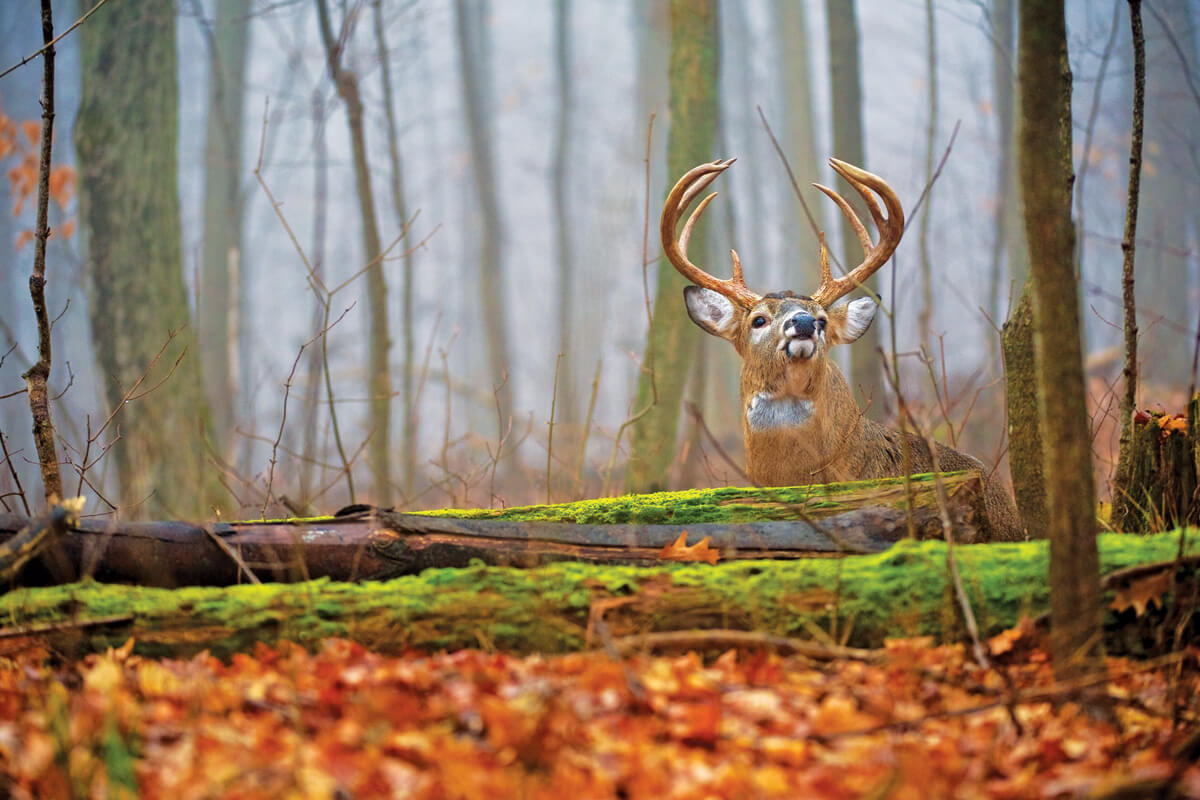In the misty forest backdrop of this vibrant, professional photograph, a large buck with impressive, curved antlers—each boasting four points—takes center stage. Its deep brown body contrasts with the striking white markings on its chest and around its mouth, while a prominent black nose adds definition to its regal profile. The deer navigates behind fallen logs on the forest floor, which are lush with neon-green moss. The ground is carpeted in a rich tapestry of red and brown leaves, indicative of fall. The trees in the background stand bare, shrouded in a soft, ethereal mist that enhances the cool, serene morning ambiance. The entire scene is an exquisite interplay of colors and textures, capturing the serene beauty of nature with exceptional clarity and depth.